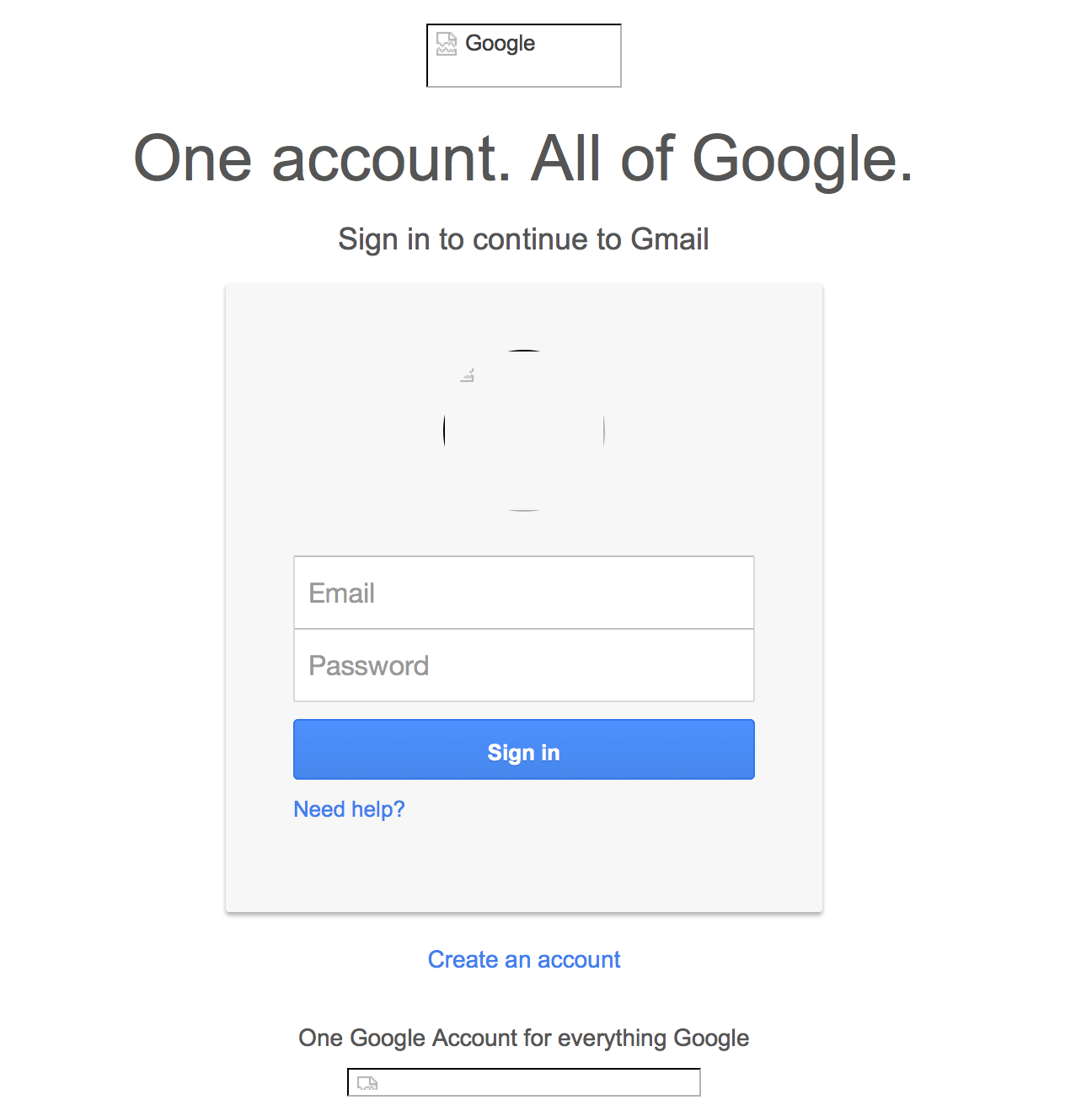The image depicts a classic Google sign-in page set against a white background. At the top, bold text reads "Sign in to continue to Gmail," indicating the purpose of this login screen. Below this heading is a square containing the colorful Google logo.

The primary section of the page is a light gray box containing two input fields: one labeled "Email" and the other "Password." Below these fields, there's a prominent blue button with the text "Sign In" in white font. 

Beneath the sign-in section, there are additional options "Need help?" and "Create an account" in blue text, offering assistance and the choice to establish a new Google account, respectively. 

Lastly, a line of text at the bottom reads, "One Google Account for everything Google," emphasizing the unified nature of Google's services. On the left side of the gray input box, there is an outline resembling a truck, adding an unexpected visual element to the otherwise functional design.